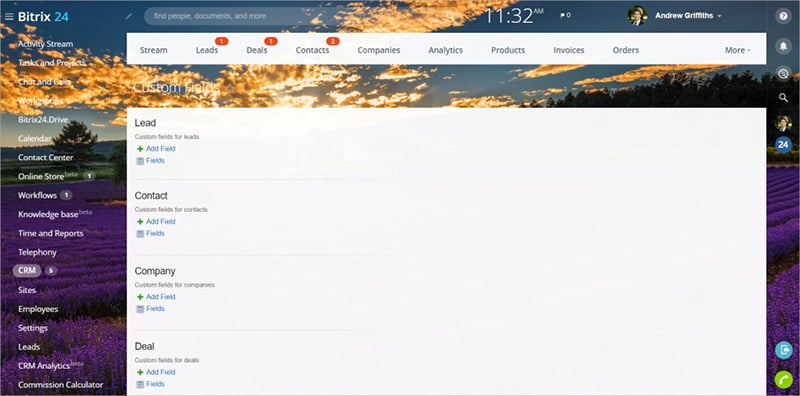This is a detailed description of a landscape-oriented screenshot depicting an application or website interface, captured against a vivid blue sky adorned with sunlit, yellow-tinged clouds. The image dimensions are approximately one and a half times wider than its height. Below the sky, there are fields of vibrant purple violets adding a splash of color to the scene.

In the top left corner of the interface, a white hamburger menu is visible, followed by the name "Bitrix24," with "Bitrix" in white and "24" in light blue letters. Adjacent to this, a grey text bubble features the query "Find people, documents, and more," along with the time "11:32 a.m." An avatar of a man dressed in a suit is next to it, labeled "Andrew Griffiths" in white text.

The left side of the interface displays a vertical navigation bar, listing various options such as "Activity Center," "Tasks and Projects," "Bitrix Drive," "Calendar," and "Contact Center," some of which have white notification icons beside them.

Occupying the central portion of the interface is a lengthy, rectangular white box with the word "Lead" prominently displayed. This section includes blue links for "Add Field" and "Fields Options," along with corresponding icons. Below this, options for "Contacts," "Company," and "Deal" are presented, each allowing customization and the addition of fields.

On the right side, the interface is bordered by icons for a phone, notifications, and a question mark, providing quick access to these functions.